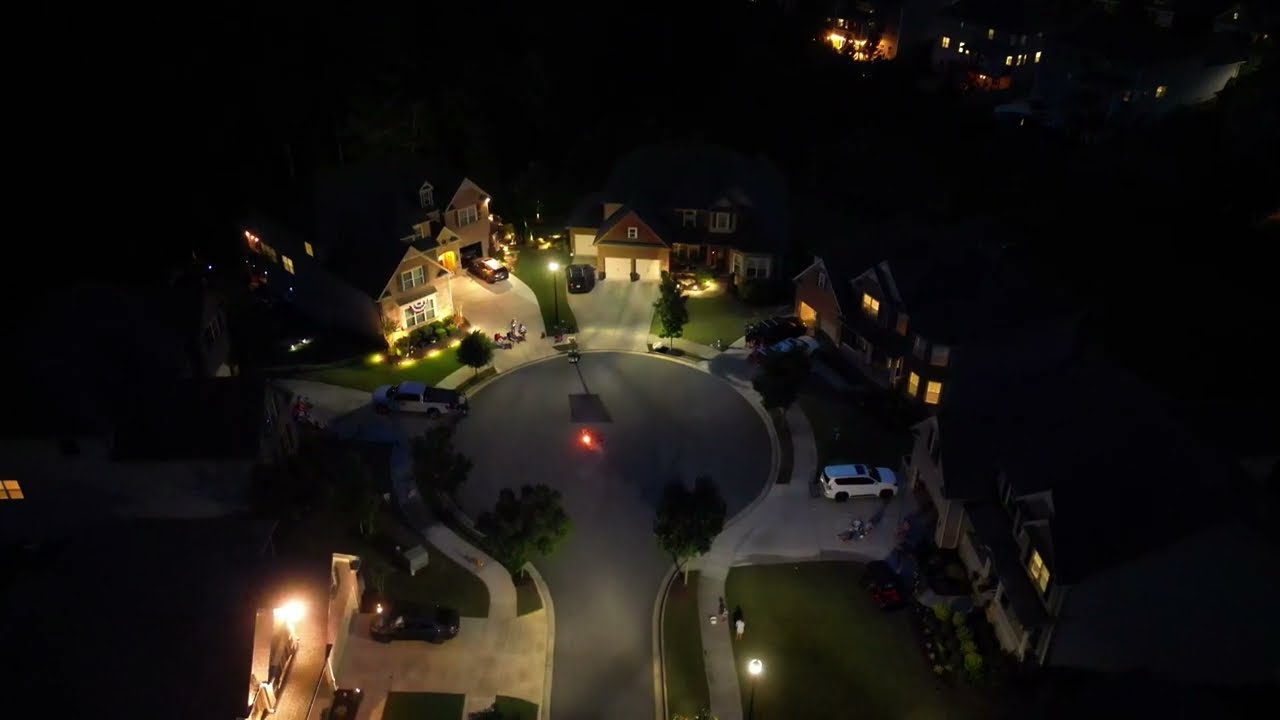The aerial, nighttime image captures a serene suburban cul-de-sac. At the center of the image is a perfectly circular road bordered by a neatly paved light gray sidewalk and verdant, freshly mowed lawns. The road, leading up to the circle from the middle bottom of the image, is paved in gray and flanked by towering green trees. Behind the trees stand large, multi-story brown houses, each with numerous glowing windows and long light gray driveways that harmonize with the surrounding sidewalk.

In the center of the roundabout, a solitary red light shines brightly, accompanied by several yellow lampposts that cast a warm glow on the sidewalk. The night sky is a deep, uninterrupted black, accentuating the peaceful atmosphere.

Several residents are enjoying the pleasant evening; a group of three to four people is gathered in one of the brightly lit driveways, seated in chairs, and conversing animatedly. Additional figures are visible in the scene—one person is seen taking a stroll through their yard, while others sit in their driveways, enjoying the calm night. The driveways are occupied by various vehicles, including white pickup trucks and SUVs.

The image also subtly captures some streetlights on the pavement, illuminating the outer circle with a comforting glow. Though primarily dark, the outer areas of the image include specks of light from other buildings, adding to the overall charm of this nighttime suburban landscape.